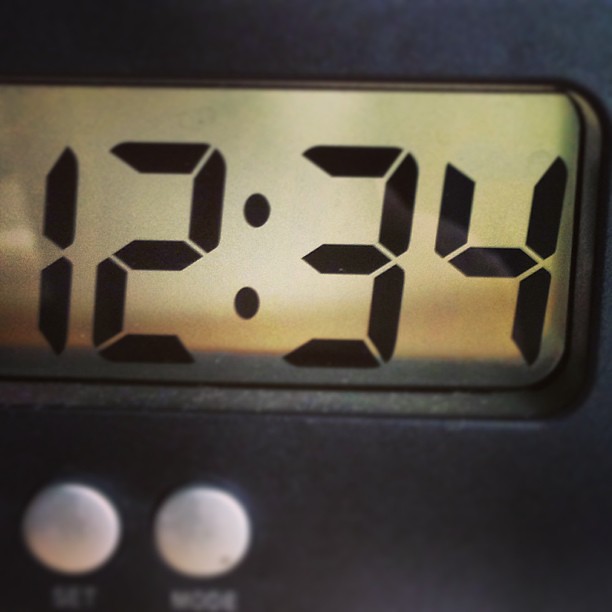This close-up, square-shaped photograph captures a black alarm clock with sleek, silver buttons. Two of these buttons are visible in the bottom left corner. The clock features a rectangular display that spans horizontally, showing the time as "12:34". The screen itself is a yellowish tan hue, while the numbers are black with a slightly pixelated appearance, lending a retro feel to the digital display.